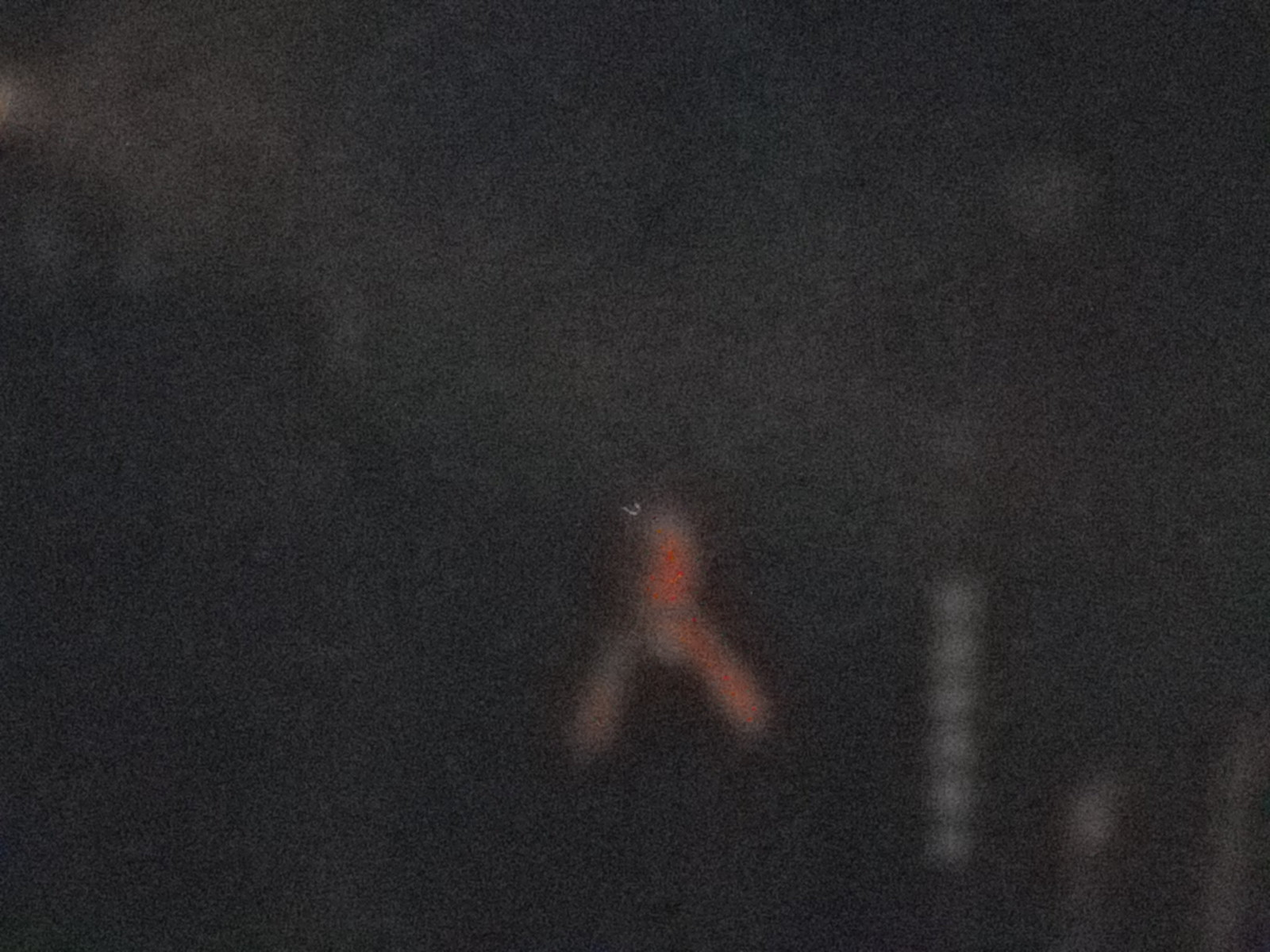Displayed in the image is a stark black and grey background with ominous, cloud-like formations that contribute to its moody atmosphere. Dominating the center is a vivid orange circular dot, drawing immediate attention and creating a striking contrast against the dark backdrop. Towards the bottom-right corner, there is a notable bright white spot. Additionally, an orange triangular shape is discernible, adding another layer of geometric intrigue to the scene. The overall composition is both minimalistic and visually compelling, with the sharp colors and shapes standing out prominently against the muted, cloudy background.